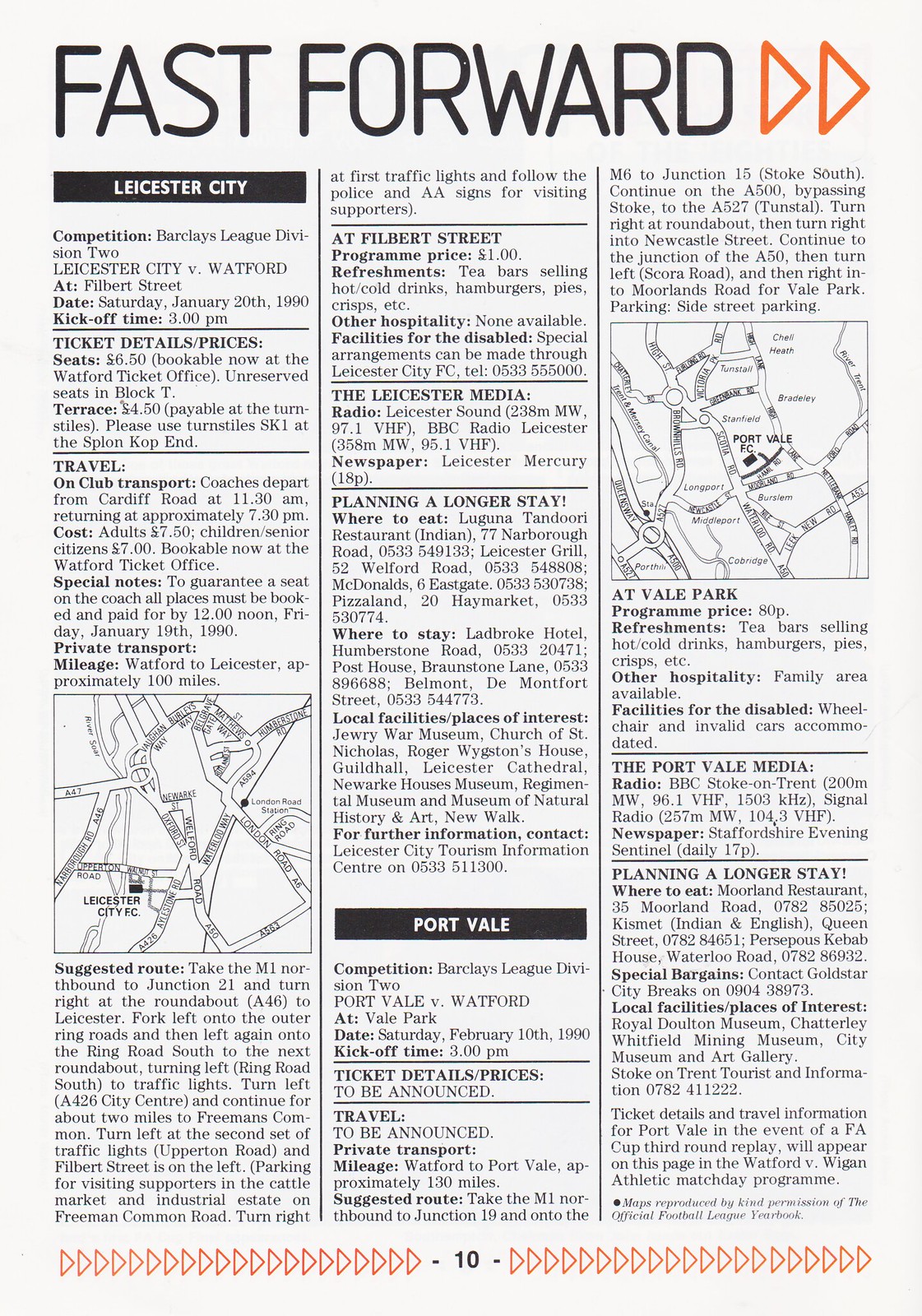This tall, rectangular image features page 10 of a light gray newspaper or game day program. At the top, bold black letters spell out "FAST FORWARD" with two orange triangles pointing to the right. The page consists of three columns. The first column is headed by a black rectangle filled with bold white letters reading "Leicester City." Below this title, various sections detailing competition information, ticket details, travel information, and points of interest are separated by horizontal black lines. A map is positioned at the bottom left of the first column. The third column mirrors this layout, featuring similar maps and detailed segments. Centrally placed at the bottom of the page is the large black number 10, flanked by rows of orange triangles pointing right. Additional details include: Barclays League Division Two, Leicester City versus Watford at Filbert Street, set for Saturday, June 20th, 1990, with tickets priced at $6.50 and available at the Watford ticket office.